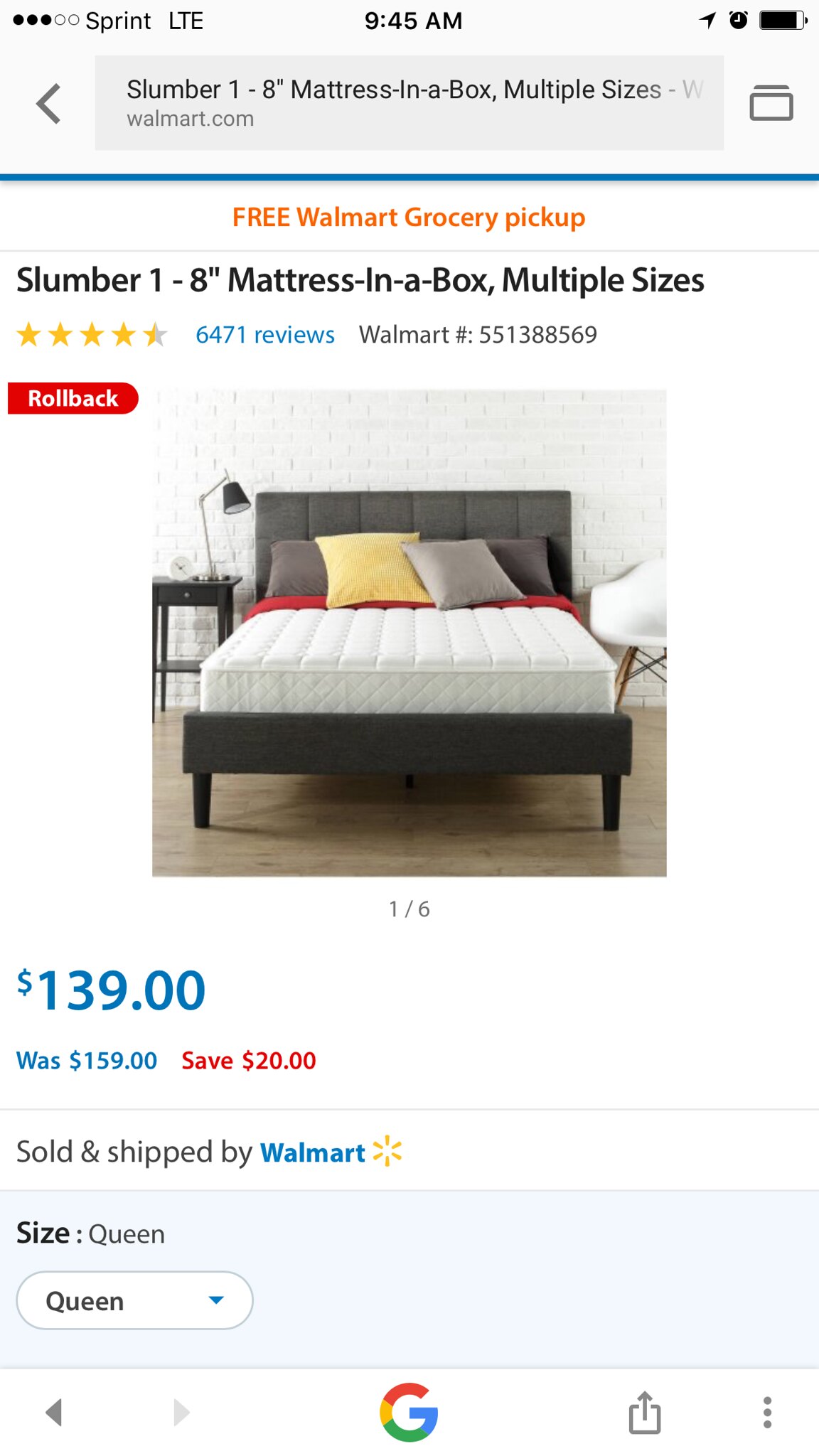This is a screenshot from an Android device showing a Walmart webpage for a "Slumber 1-8 Inch Mattress in a Box" with multiple sizes available. The device’s status bar at the top indicates it is 9:45 a.m., the carrier is Sprint with three out of five bars of signal strength, and the battery is almost full. The webpage features a detailed product listing with 64,711 reviews. The mattress is priced at $139 in blue font, discounted from its original price of $159, highlighted by a red "Save $20" label. The selected size is Queen. The visual depiction includes a photo of a grey bed with yellow and grey pillows, set against a white background, and a nightstand placed on a wooden floor. The webpage also mentions free Walmart grocery pickup and includes a drop-down menu for selecting different sizes. At the bottom, the Google logo and Android navigation buttons are visible.